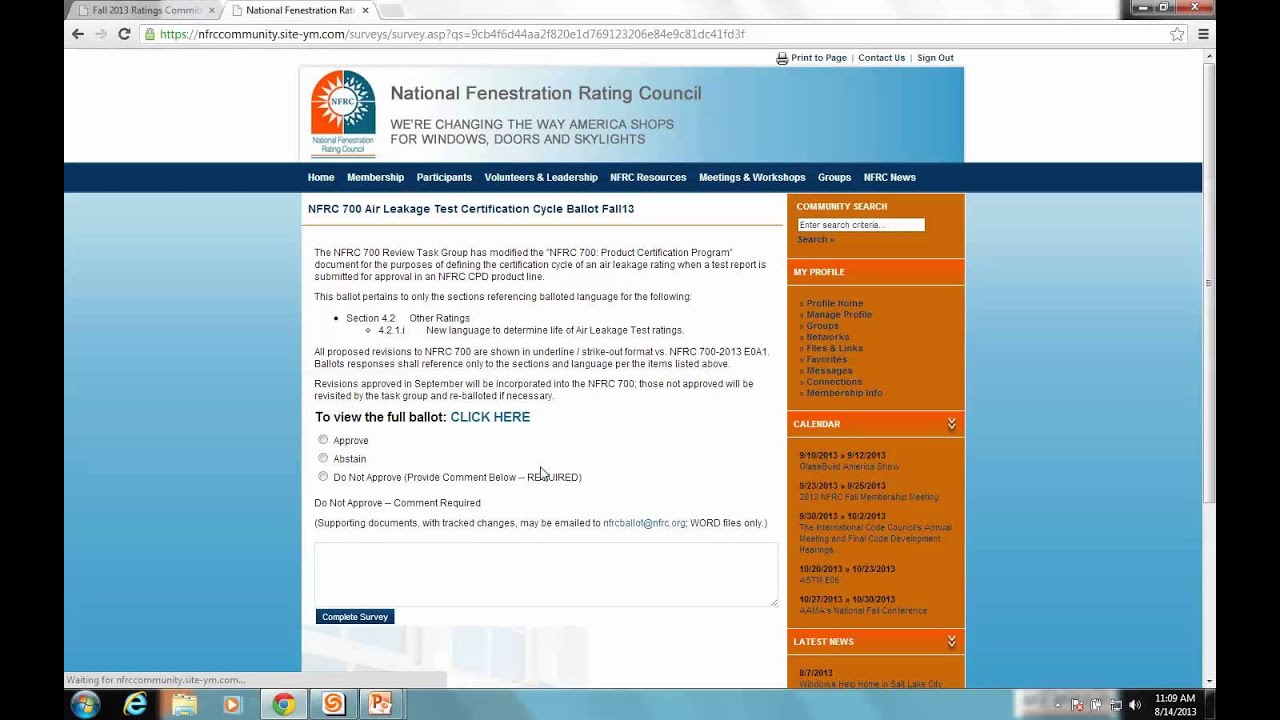This image captures a web page displayed on a computer screen, focusing on the National Fenestration Rating Council (NFRC) site. At the top of the browser, two tabs are visible. One of them, which is currently active, is labeled "National Fenestration Rating Council." The URL for the site is visible, alongside the customary 'X' button to close the tab. The screen background on either side of the web page is black, framing the central content.

The web page itself has a white background at the top, with a white border on the left and a gradient that transitions from white to blue on the right. The NFRC logo is prominently displayed on the top left corner. The logo consists of a rounded window design with orange on the left half, blue on the right half, and a white sun icon in the center. Directly beneath the logo, a tagline reads, "Changing the way America shops for windows, doors, and skylights."

Highlighted sections include headings such as "Print," "Home," "Membership," and "Participants" in blue text on a white background. Below these headings, a line of text reads, "NFRC 700 Air Leakage Test Certification Cycle, Ballot, Fall 13," followed by a dense block of writing. A prompt, "To view the full ballot, click here," appears further down the page with associated radio buttons.

On the right side of the page, an orange vertical bar features a search bar labeled "Search," followed by a "My Profile" section and various other options. Beneath this, another heading introduces additional choices. The bottom section of the page features a "Latest News" heading with several items listed underneath.

Overall, the page is organized and detailed, providing specific sections for user interaction and additional information.